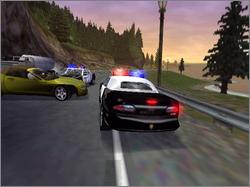This image is a pixelated screenshot from a dated video game, possibly an adventure or racing game akin to Grand Theft Auto. The scene is set outdoors on a gray road with a white vertical stripe, one lane going in each direction, and it captures the dynamic tension of a police chase. Dominating the center is a police car with a white roof and red rear, equipped with flashing red and blue lights on top. The car appears to be braking, yet its left brake light is malfunctioning. Nearby, a yellow-green convertible is oriented at a sharp angle to the police car, hinting at a collision or evasive maneuver. Another police car follows, intensifying the chase. The left side of the frame reveals scattered equipment or perhaps a tank on the roadside. The environment includes a coniferous landscape: to the right, a solitary fir tree stands next to a pole light featuring a yellow torch-like light, behind which lies a grassy area leading to a likely body of water. Ahead, a forest of conifer trees crowns a steep, rocky hill. The image, though dated, vividly portrays a moment of high action and pursuit.